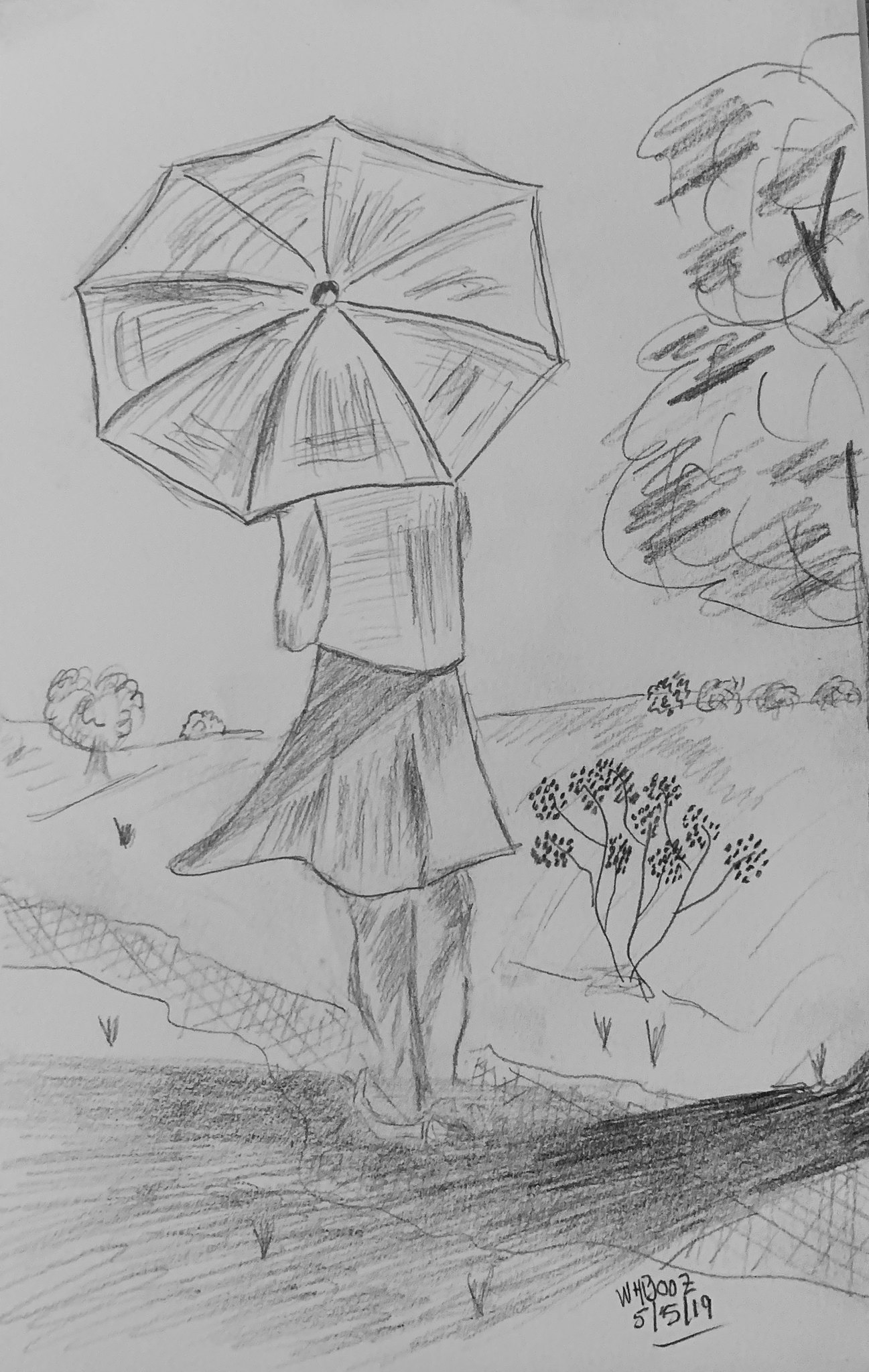A detailed charcoal or pencil sketch, dated May 5th, 2019, captures the serene and slightly surreal scene of a woman standing in a small stream. The artist's signature is visible on the artwork. Dominating the composition, the woman appears as a giant, dwarfing the rolling hills and trees that stretch out in the distant background. Viewed from behind, she seems to be either barefoot or wearing flats. A slight breeze lifts the mid-thigh length skirt she is wearing, causing it to waft gently to the left. Her long-sleeved shirt or blouse adds to her somewhat enigmatic appearance. Intriguingly, the woman's head and the upper part of her shoulders are concealed by an open umbrella she holds, adding a touch of mystery to her identity. To her right, another tree is depicted, in proportion to her giant stature, reinforcing the whimsical and rough sketch style, all set against a stark white backdrop.